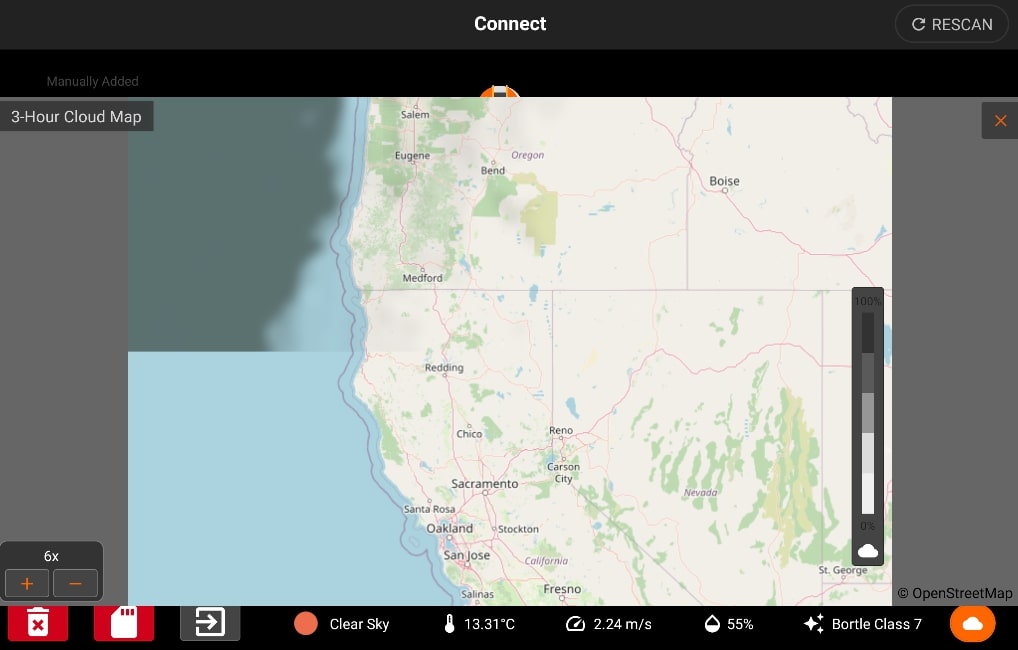Detailed Caption: 

The image is divided into several sections, each featuring specific graphical elements and text. 

At the top and bottom of the image, there are dark gray bands, creating a frame-like effect. In the center, there's a prominent, white-colored text that reads "CONNECT" in all capital letters. Directly below this text is a gray oval containing a white arrow that forms a circular shape, resembling a refresh button. 

To the right of this gray oval, there's the word "RESCAN" also in capital letters, indicating another interactive option.

In the lower part of the image, there are two red squares. The first red square features a white icon of a trash can, suggesting a delete option. Adjacent to it, the second red square displays a white letter icon, likely representing a messaging or mail function.

Next to these, there's a gray square with a white arrow pointing to the right, hinting at a forward or next action. 

Further along, there's a yellowish-orange circle with the text "CLEAR SKY" in white, indicating the current weather condition. Adjacent to this circle, there's a white thermostat icon followed by the text "13.31°C" in white, denoting the temperature. 

Nearby, a white meter-like icon is shown with the accompanying text "2.24 m/s" in white, likely indicating wind speed. Next to this, another icon resembling a water droplet is displayed along with the text "55%" in white, representing humidity levels.

Additionally, there are three white stars followed by the text "Portal Class 7," indicating a rating or classification.

An orange circle with a white cloud icon signifies weather details. Above this section, there's a black "C" within a circle, symbolizing copyright, and the text "OpenStreetMap" in black, referring to the map source.

The map itself is displayed below, showing various labels: "Oregon" in the upper region, "Oregon Boys" slightly below, "Nevada" to the right, with "Chico," "Reno," "Carson City," "San Jose," and "Oakland" placed towards the central areas, followed by "Fresno," "California," and "St. George" further down. The map also features a significant water body on its left-hand side.